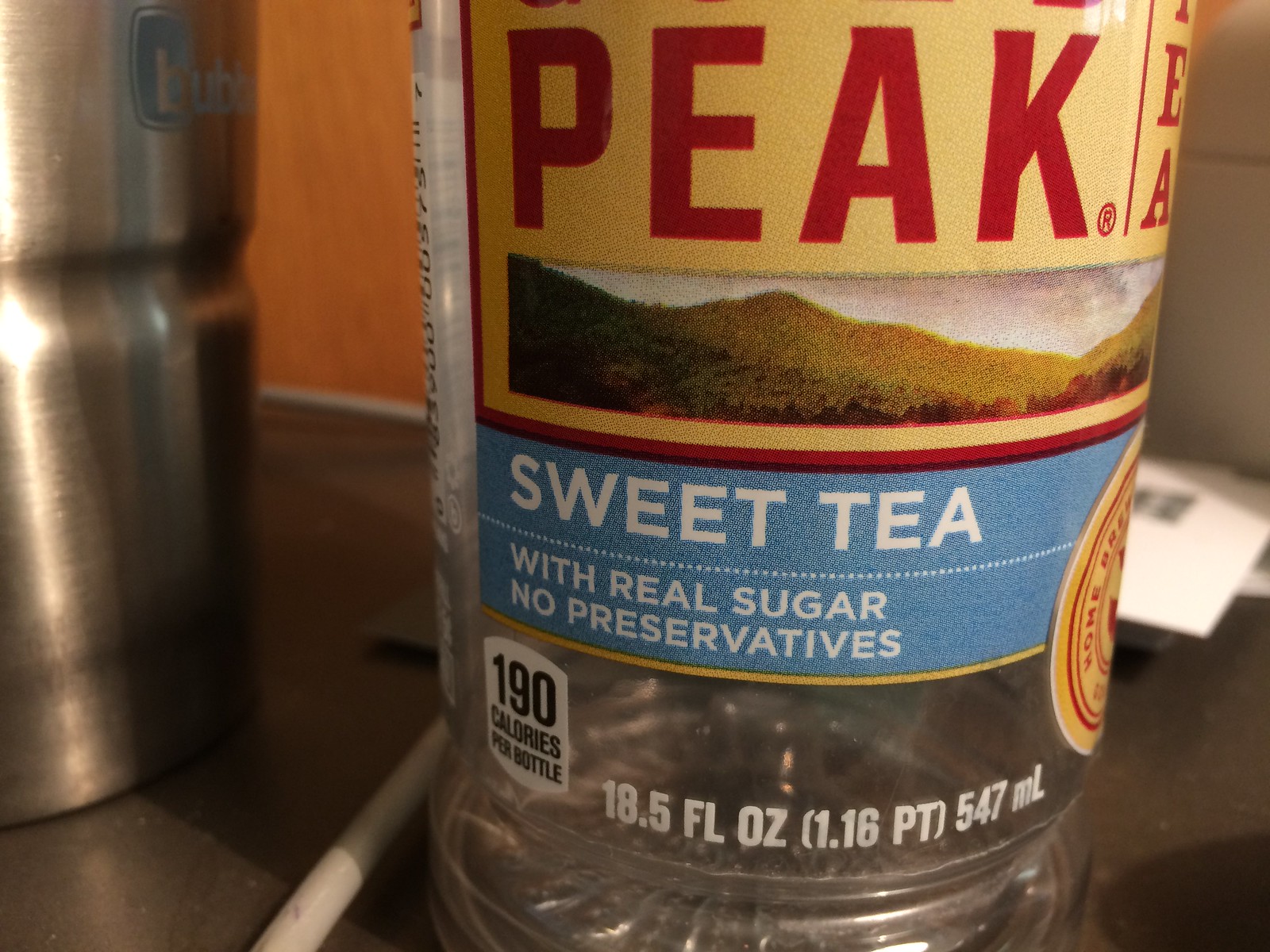This close-up photograph captures a detailed view of a gold-labeled sweet tea bottle from the brand "Gold Peak." At the top of the label is the word "PEAK" in bold red text, with an image of a valley beneath it. The label reads "Sweet Tea with Real Sugar, No Preservatives" on a blue background with white text. The bottle also lists its nutritional information as "190 calories per bottle" and specifies the volume as "18.5 fl oz, 1.16 pt, 547 ml." The bottom right corner features a seal indicating the tea's freshness. The bottle appears empty and is positioned on a silvery, matte grey desk surface. To the left of the tea bottle is a silver thermocup with partially visible text, appearing to show the letters "CUBI" in light blue. Behind the bottle, one can spot the top of a barcode and some envelopes or mail scattered on the desk. The background includes an orange wall and tiles. The main focus of the image is the detailed label on the Gold Peak sweet tea bottle.